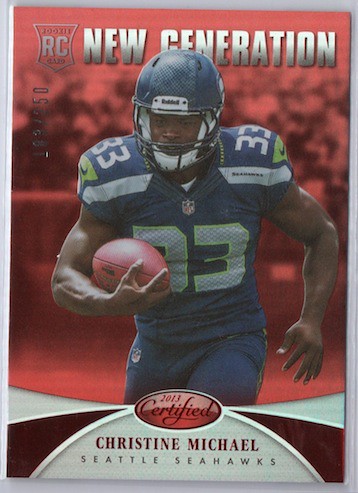The image appears to be a football card featuring a Seattle Seahawks player. At the top, a bright red background displays an emblem with the letters "RC" and the words "New Generation" in white. Centrally positioned is an African-American football player, identified as Christine Michael, wearing the number 33. He is captured in motion, running with a football clutched in his right arm and his left arm positioned near his body. His uniform includes a blue helmet, blue pants, and a blue shirt adorned with light green accents and gray stripes. The background, filled with white specks indicating an indistinct crowd, adds to the dynamic feel of the card. At the bottom, a red circle within a white banner reads "2013 Certified Christine Michael Seattle Seahawks." The overall color scheme features a rich variety of hues including red, black, white, gray, various shades of blue, lime green, maroon, and a vibrant orange football. This card highlights and promotes Christine Michael and his affiliation with the Seattle Seahawks.